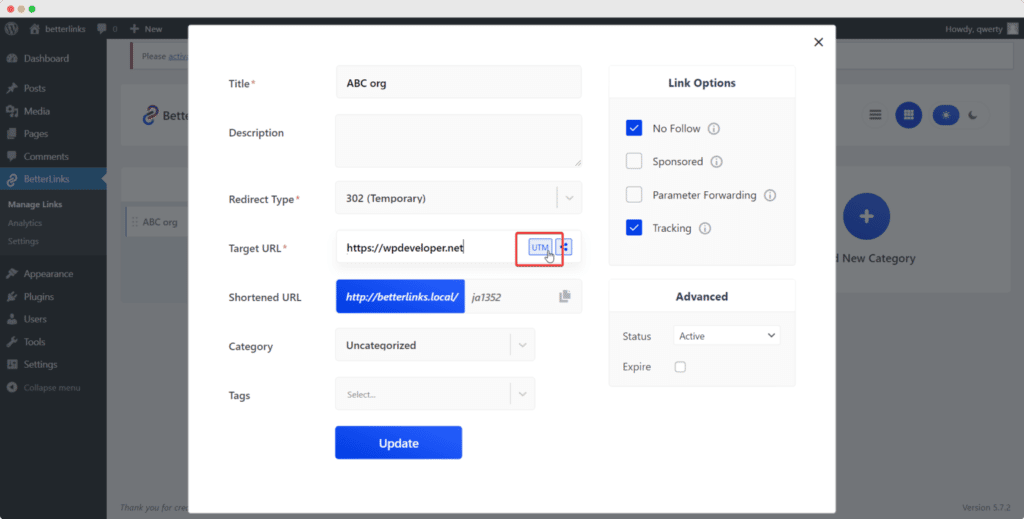A detailed caption for the described image could be:

"A user is working on a WordPress site, as evidenced by the familiar W logo in the upper left corner of the screen. The developer is using a Macintosh computer, identifiable by the colored icons in the upper left of the window. The dashboard menu on the left side lists various sections such as Posts, Media, Pages, Comments, Better Links, Plugins, Users, Tools, and Settings. The user is currently in the 'Better Links' section, indicated by the blue highlight. 

The interface displayed includes fields and options for configuring a link. The 'Title' field is set to 'abc.org', and next to it are options for adding a description (currently left blank) and specifying a 'Redirect Type', which is set to '302 Temporary'. The 'Target URL' field contains 'https://wpdevelopers.net', and the 'Shortened URL' field shows 'betterlinks.local.j01352', displayed as a blue button.

Further down, the category is set to 'Uncategorized', with a prompt to select tags, and there's an 'Update' button at the bottom. To the right of the 'Target URL' field is a callout area highlighted in red, with a cursor area labeled 'UTM'. A vertical menu labeled 'Link Options' features settings like 'No Follow', 'Sponsored', 'Parameter Forwarding', and 'Tracking', with 'No Follow' and 'Tracking' currently selected. Beneath these options is an 'Advanced' section with 'Status' settings, where 'Active' and 'Expire' are available but not selected."